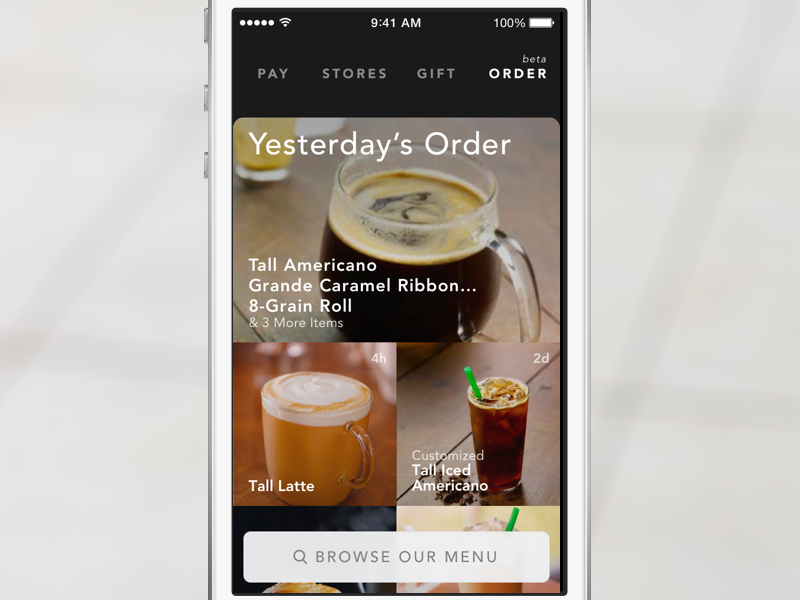The image showcases a white smartphone with a gray background. The smartphone screen displays the time as 9:41 a.m. and shows a fully charged battery at 100%. The screen also features an application interface with highlighted text reading "Pay, Stores, Gift, and Order." The "Order" section is selected, revealing details of "Yesterday's order," which includes items such as a Tall Americano, a Grande Caramel Ribbon Crunch, an Eight Grain Roll, and three additional unspecified items.

Placed on a brown wooden tabletop, the clear glass mug in the foreground has a handle and contains a brown liquid with a slight foam on top. Partially visible behind this mug is another cup, though only a portion of it is discernible. Beneath these, a clear cup filled with foam and sprinkled with what appears to be cinnamon is labeled as a "Tall Latte." Additionally, there is a tall glass filled with ice and brown liquid, identified as a "Tall Iced Americano."

At the bottom of the screen, a button prompts users to "Browse our menu."